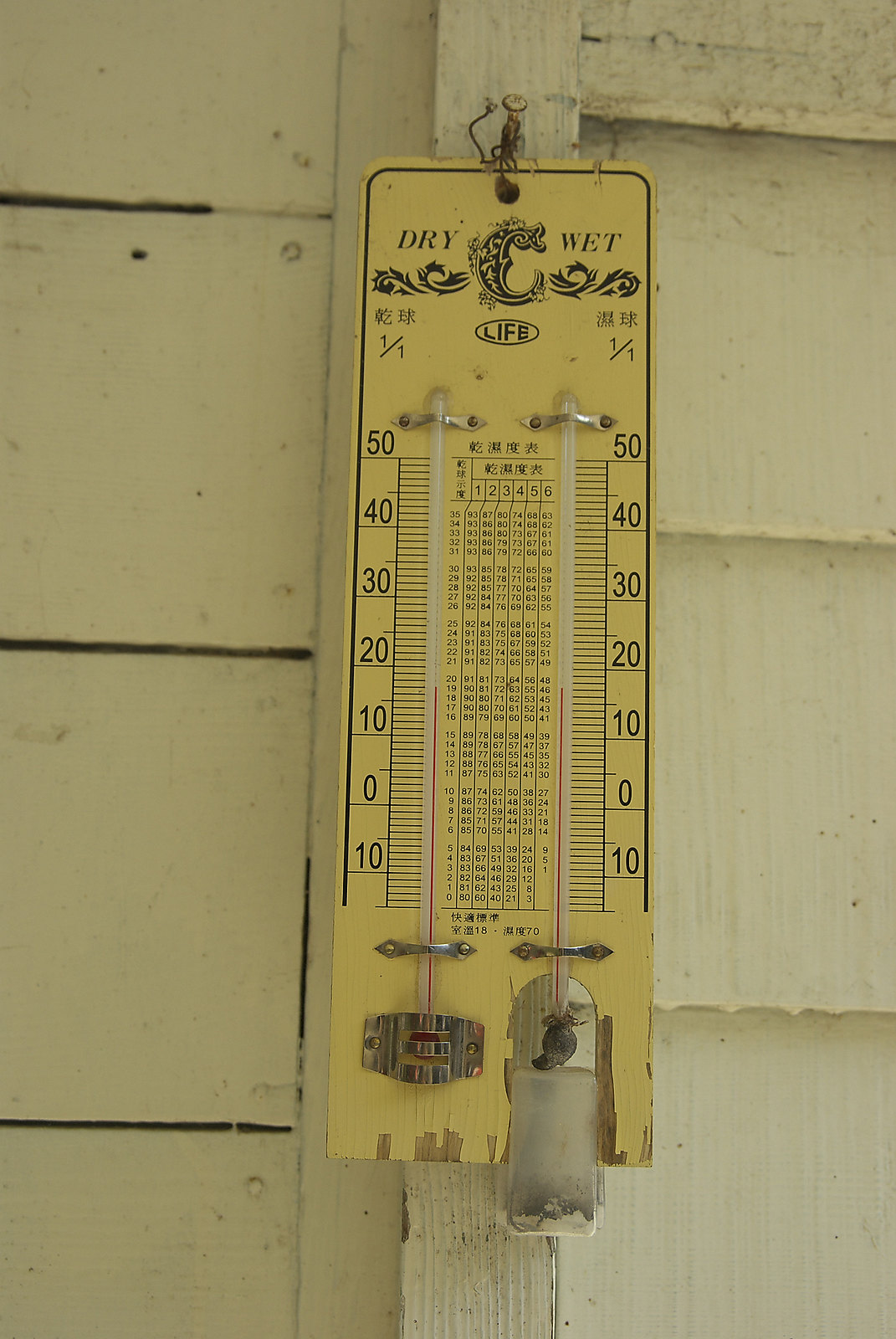A rustic, weathered house with a wooden exterior that resembles a barn is the focal point of this outdoor scene. The structure shows signs of age and wear, adding character to its appearance. Affixed to a protruding nail on the wall is an intriguing dual thermometer. This unique measuring tool displays identical temperature scales on both sides, ranging from 50°F down to -10°F and back up to 10°F. The left thermometer appears securely in place, while the right one is held together with a makeshift metal bracket, suggesting a repair job.

The thermometers are mounted on a yellow-painted wooden board, which exhibits chipped paint, revealing the underlying wood. The central section of the board is densely packed with various numbers and four columns of data. The middle displays a sequence from 1 through 6 horizontally, and another vertically ascending from 0 to 35. The rightmost part of the thermometer shows readings up to 63, with other numbers scattered in between, likely indicating different temperature units or reference points. Despite the worn state of the board, the dual thermometers remain functional, adding a historical, practical element to the otherwise dilapidated façade.